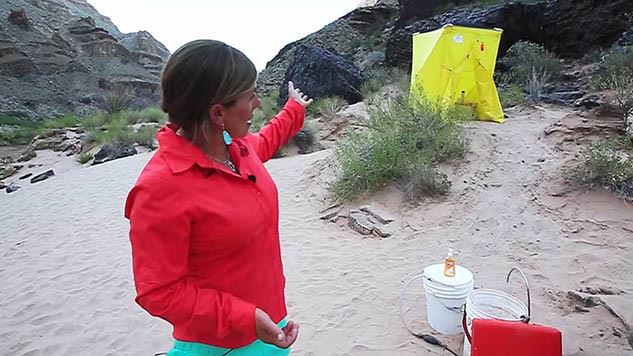In this outdoor photograph, a woman stands in a desert-like landscape with sandy ground and scattered vegetation. She is dressed in a red collared shirt and light blue pants, with dark brown hair styled short. She accents her outfit with blue tag earrings. Her left arm is outstretched in a pointing gesture, drawing attention to a yellow structure near her, which appears to be a complex tent featuring multiple triangular facets, partly obscured by a nearby bush. 

Behind the tent are imposing, dark hills framing the scene on both the left and right. The ground around her shows signs of camping activity with two white containers – one holding a bottle that looks like hand sanitizer, while the other, open, has a red object attached beside it. The setting brings to mind camping areas such as Joshua Tree, likely due to the distinctive desert foliage and terrain.